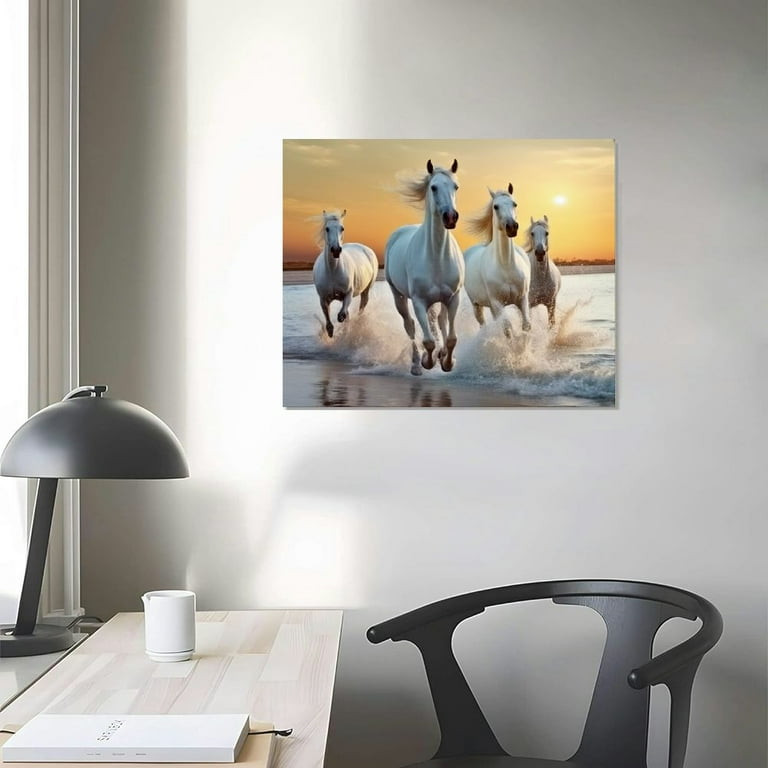The full-color, vertically rectangular photograph captures a carefully staged indoor scene illuminated by natural daylight. Dominating the composition is a vivid painting of four white horses galloping along a beach, their hooves splashing through the water as the horizon glows with an amber-orange sunset. The artwork hangs on a plain gray wall, which catches some natural light filtering through open blinds on the left side of the image. Below the painting is a wooden desk with light-colored slats, on top of which sit a black desk lamp, a white coffee mug, and a book in the lower right corner. A black chair accompanies the desk, contributing to the organized yet lively atmosphere of the scene.